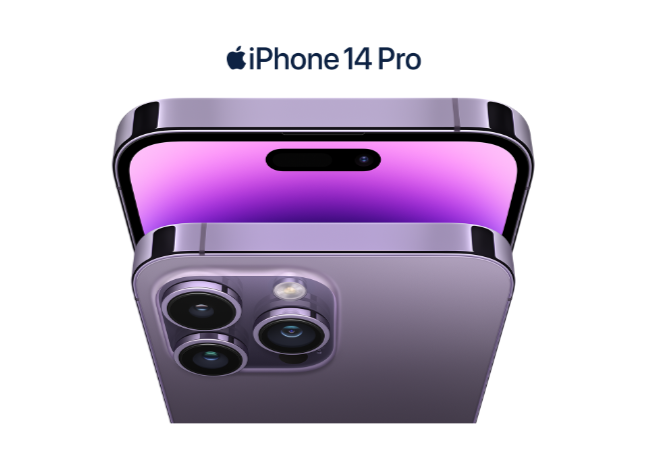In this professionally crafted advertisement for the iPhone 14 Pro, the high-quality image prominently showcases the sleek design and advanced features of the latest Apple offering. At the top of the image, the words "iPhone 14 Pro" are displayed in elegant font, accompanied by the iconic Apple logo to the left.

The image features two iPhones positioned to highlight both the front and back of the device. The upper iPhone faces the viewer, allowing a clear view of the vibrant home screen, which displays a captivating gradient background transitioning from dark purple in the center to a lighter purple towards the edges. This screen is turned on, demonstrating the device's vivid display capabilities.

Nestled against this front-facing iPhone is another device, viewed primarily from the back. This secondary iPhone is shown in an alluring gray-purple color, a hallmark of its sophisticated design. The rear of this phone highlights the advanced camera system, featuring three distinct lenses located in the upper left corner along with a visible flashlight, underscoring the phone's premium photographic capabilities.

The overall composition of the advertisement presents a compelling visual narrative, emphasizing the elegance, functionality, and innovation of the iPhone 14 Pro.